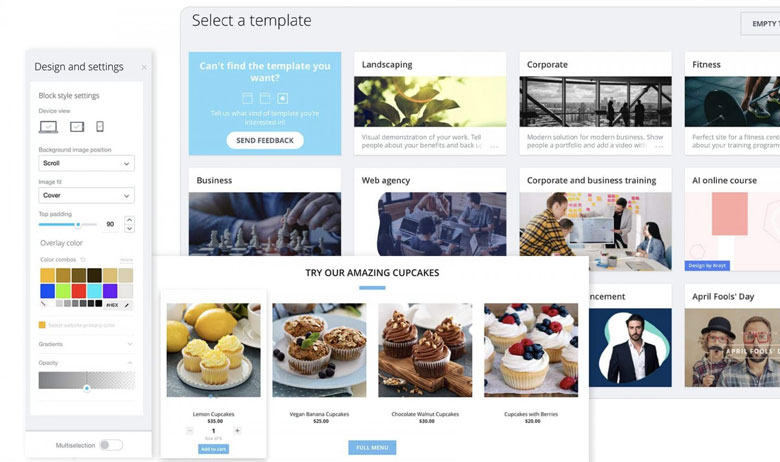This screenshot captures a photo editing website that appears highly versatile, functioning similarly to platforms like Canva, where users can choose images or layouts and customize them according to their needs. At the top of the screen, there is a section with black text that reads "Select a Template." This area features various template options including "Landscaping," "Corporate," "Fitness," "Business," "Web Agency," "Corporate and Business Training," and "AI Online Courses."

Interestingly, the bottom of the screen showcases another section that promotes cupcakes, with the text "Try our amazing cupcakes" in black. Below this text, there are images of four different types of cupcakes, each labeled accordingly: "Lemon Cupcakes," "Vegan Banana Cupcakes," "Chocolate Walnut Cupcakes," and "Cupcakes with Berries." Each cupcake image is matched with its corresponding name, and the pricing seems high, suggesting perhaps a gourmet or bulk offering at $35, $25, $30 respectively.

On the left side of the screen, there are multiple design and settings options, including features like scrolling, image fit adjustments, and overlay color modifications. This suggests that the site is geared towards providing users with extensive customization capabilities for their projects.